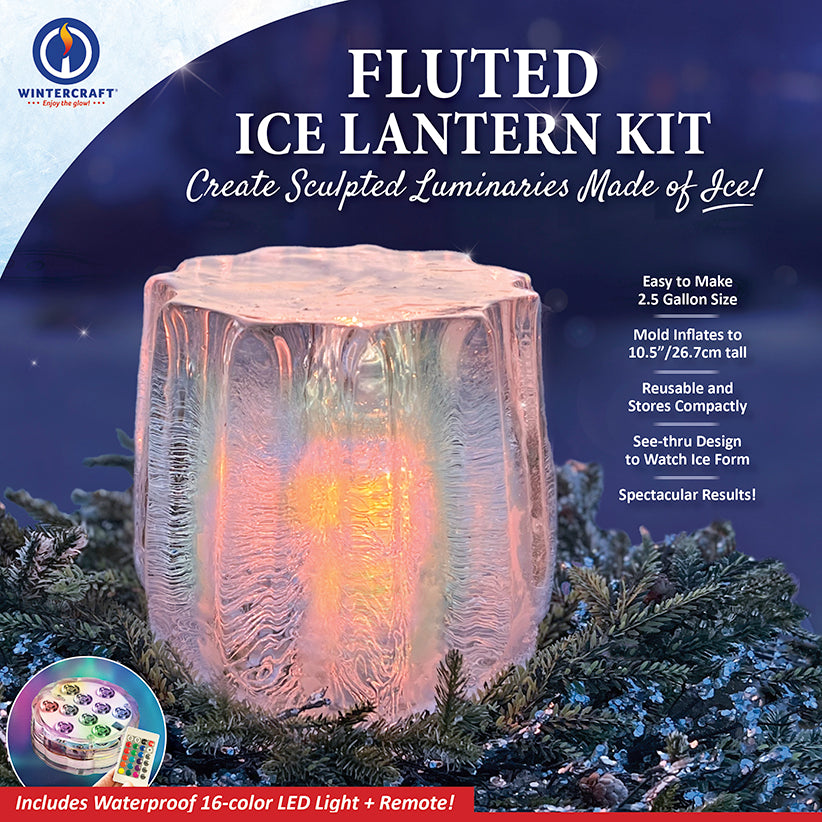The image depicts the front of a box for the Wintercraft Fluted Ice Lantern Kit, set against a backdrop of green evergreen branches. The kit allows users to create sculpted luminaries made of ice, featuring a mold that inflates to a size of 10.5 inches (26.7 cm) and holds up to 2.5 gallons. The ice lanterns are designed to be reusable and can be stored compactly. The see-through mold enables users to watch the ice form, yielding spectacular results. The kit includes a waterproof 16-color LED light and a remote control for effortless illumination. The text on the box highlights the ease of creating these ice lanterns and the enchanting glow they produce, making them an ideal decorative piece, especially during the holiday season.